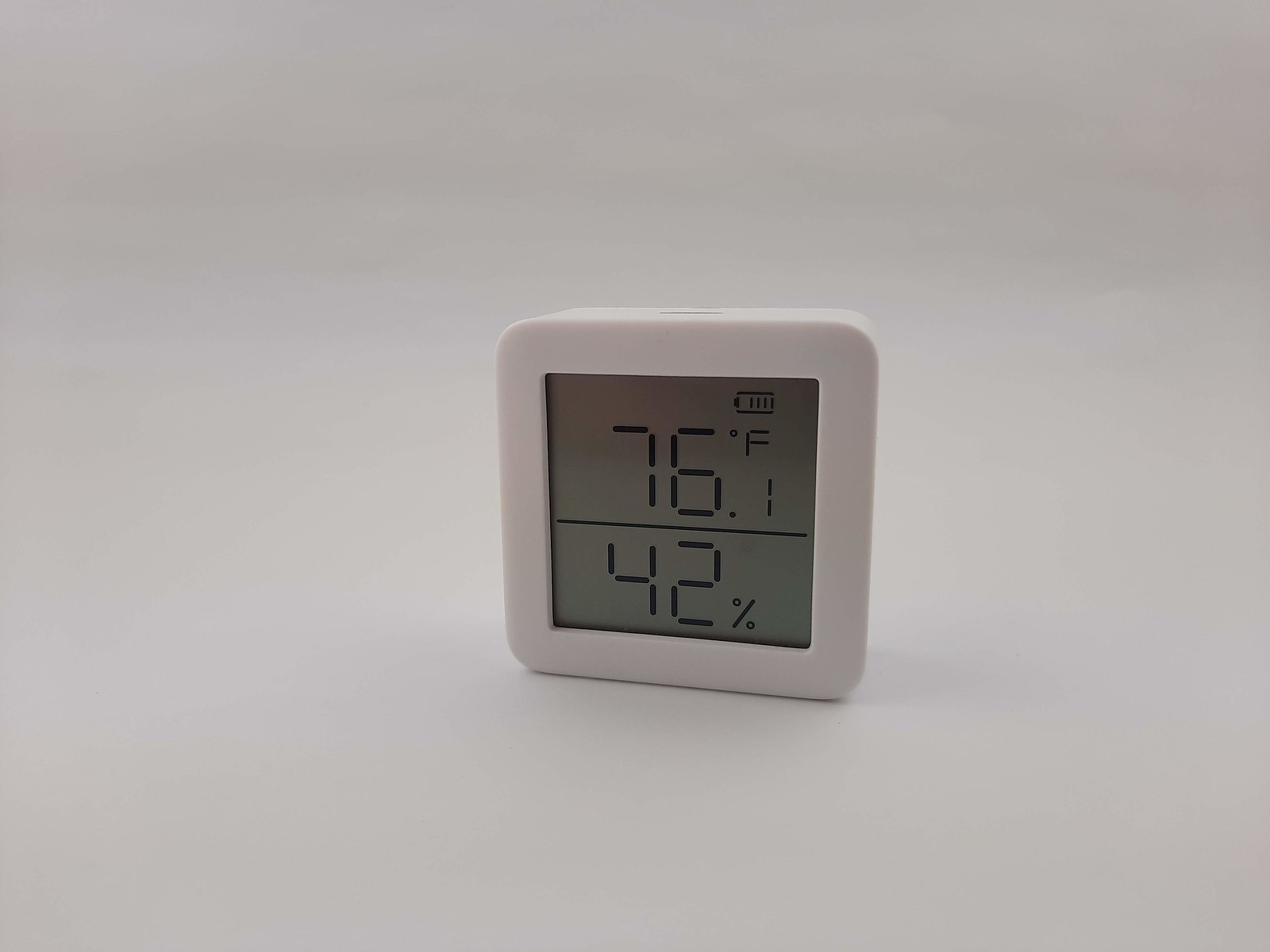The photograph showcases a compact digital thermometer and humidity gauge with a sleek white square design. The device features a clear LED display screen that uses a typical digital clock style font for easy readability. The top portion of the screen displays the battery level icon and the current temperature, which is 76.1 degrees Fahrenheit. A thin divider line separates the top display from the bottom half, which indicates the humidity level at 42%. Both temperature and humidity readings are presented in black numerals, ensuring high contrast against the light background for enhanced visibility. The entire unit is framed by a white border and is set against a matching white background, adding to its minimalist and modern aesthetic.